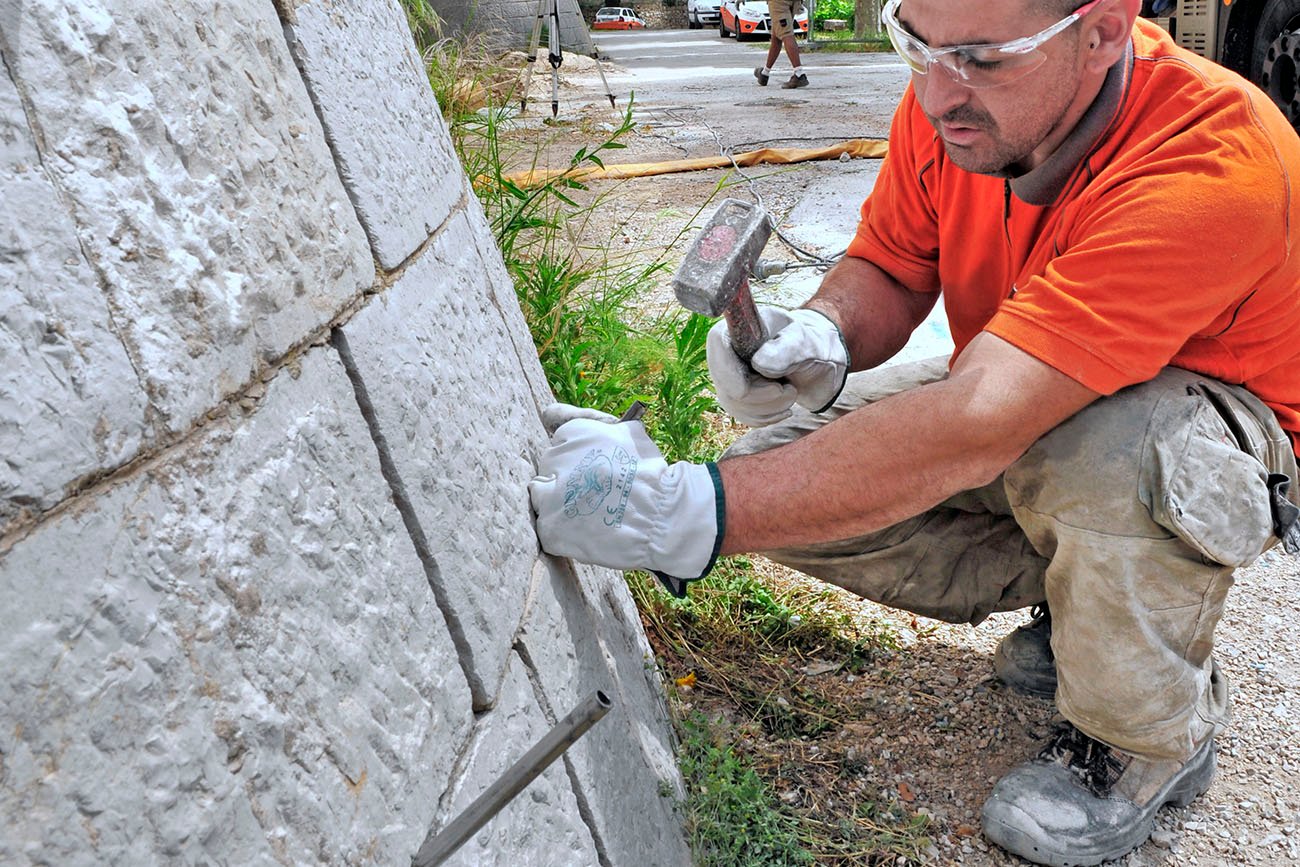The image displays a white man kneeling outdoors, meticulously working on what appears to be a gray brick wall. He is dressed in an orange shirt with a brown collar and stained tan work pants. His dirty black steel-toe boots are planted firmly on a gravel surface with some disheveled grass nearby. White work gloves with blue accents protect his hands as he wields a hammer in his right hand and a chisel in his left. Safety goggles shield his eyes from debris as he appears to be either chiseling or repairing the wall. The scene is set in a yard or street with a small hose on the ground and three vehicles in the background—one white and two with an orange bottom and white top. In the background, an individual wearing black shoes walks away from the scene, perhaps another utility worker. The overall setting suggests a detailed focus on the man's meticulous and labor-intensive work outdoors.